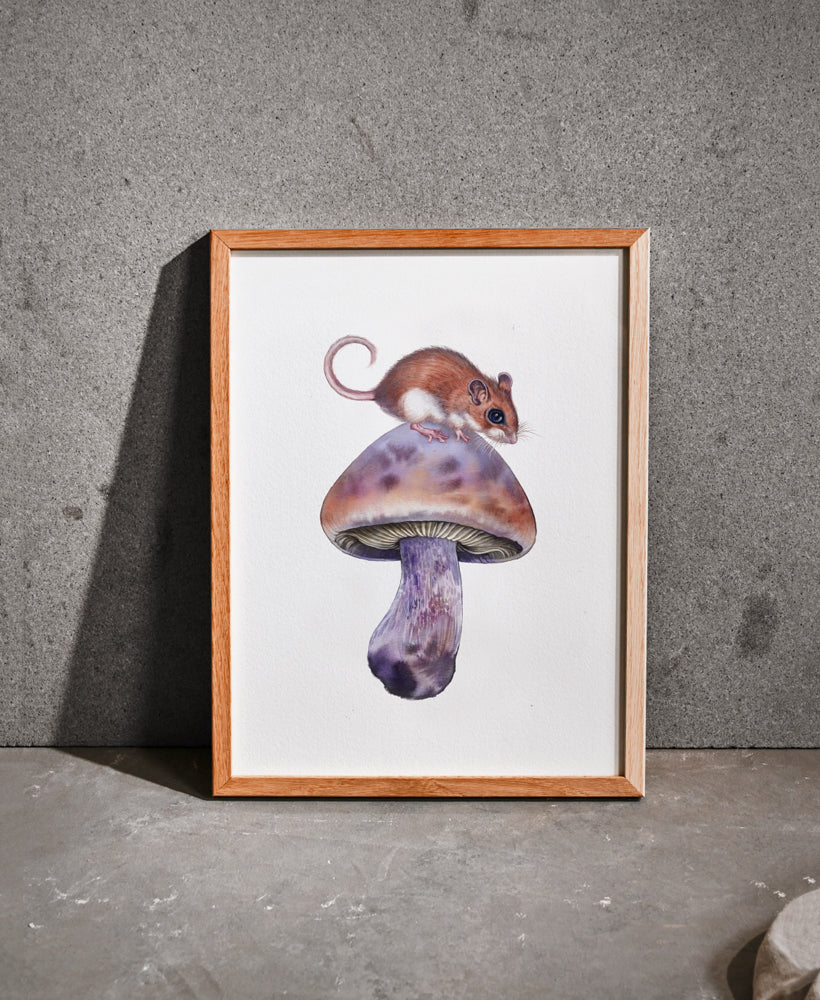This framed drawing, set against a gray concrete wall and resting on a gray concrete surface, vividly captures a charming scene with a meticulous level of detail. The artwork itself is surrounded by a dark tan wooden frame, and its background is a bright, solid white. The central focus is a brown field mouse with a distinctive white belly and a white patch beneath its mouth. It sports rounded ears, a tapered nose, black whiskers, and a large black eye, adding a touch of realism to its endearing appearance. The mouse’s curly tail forms a perfect 'C' shape. Perched gracefully on all fours, the mouse sits atop a toadstool that’s primarily light brown with brown spots and white ridges visible on its underside. The stem of the toadstool features a complex pattern of gray with brown splotches. While the exact colors of the mushroom vary in the descriptions, including mentions of purple, black, and tan hues, the toadstool presents an intriguingly colorful base for the mouse. Sunlight casts a subtle shadow on the back wall, suggesting the photograph was taken in natural light. In the bottom right-hand corner of the image, the edge of a circular object, possibly the base of something like a piece of furniture or another decorative item, can be seen peeking into the frame.